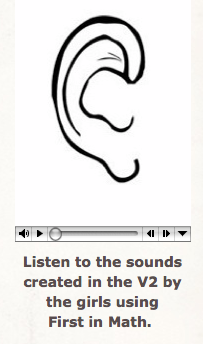The image is a tall rectangular screenshot of a computer application, featuring a black ink drawing of an ear in profile on a white background. Below the ear, a silver progress bar spans across the width of the image. This bar includes a volume symbol, play button, progress indicator, rewind button, and fast-forward button. Underneath the bar, in dark gray or brown text against a light gray or beige background, the caption reads: "Listen to the sounds created in the V2 by the girls using First in Math." The text is not arranged symmetrically, varying in width from widest to narrowest.